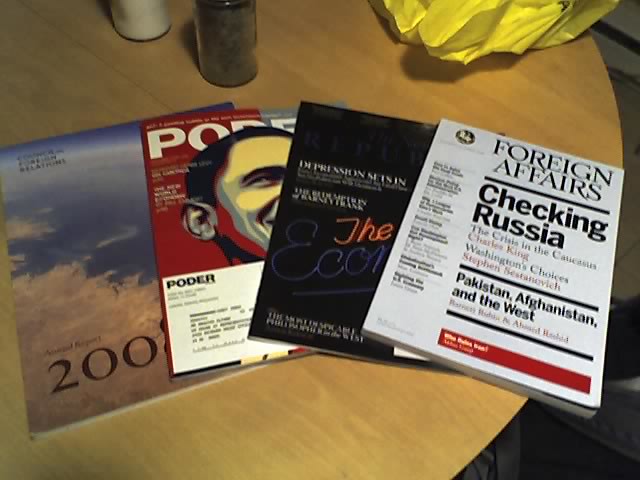This is a color photograph, slightly out of focus, capturing a horizontal, rectangular snapshot of a round, light wood-colored kitchen table. The table hosts an assortment of items, prominently featuring four magazines. Toward the left edge of the frame, partially obscured, are a pair of salt and pepper shakers. Of the magazines, one, positioned prominently, is titled "Foreign Affairs" and has a cover story on "Checking Russia, Pakistan, Afghanistan, and the West." Adjacent to it is a black-capped magazine, likely "The Economist," with a cover headline mentioning "Depression sets in." Another magazine, "Poder," displays a graphic arts portrait of former President Obama on its cover. The fourth magazine is an annual report with a partially obscured date, presumably from the early 2000s. Additionally, there is a noticeable piece of yellow material or paper on the table. The composition and thematic content of the magazines suggest a focus on world events and political affairs from around the late 2000s.